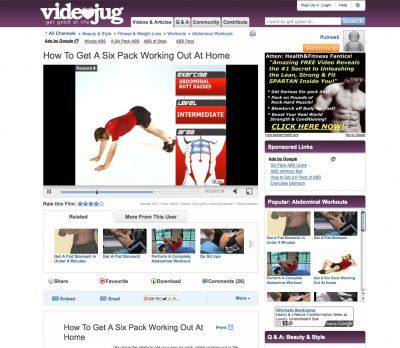On a website called VideoJug, where the 'O' in 'Video' is creatively shaped like a heart, a paused video titled "How to Get a Six-Pack Working Out at Home" is prominently displayed. The video features a Caucasian man wearing a white shirt, black shorts, and black shoes, transitioning from a downward dog yoga pose into another exercise position. The screen labels the exercise as "Abdominal Raises" or "Butt Raises," categorized at an intermediate difficulty level. An illustration highlights the upper core muscles targeted by the workout. Below the video, a section for user ratings shows the video has received 4 out of 5 stars. Accompanying the main content is a sidebar showcasing a series of related workout videos and an advertisement urging viewers to click for more exercise or health-related content.